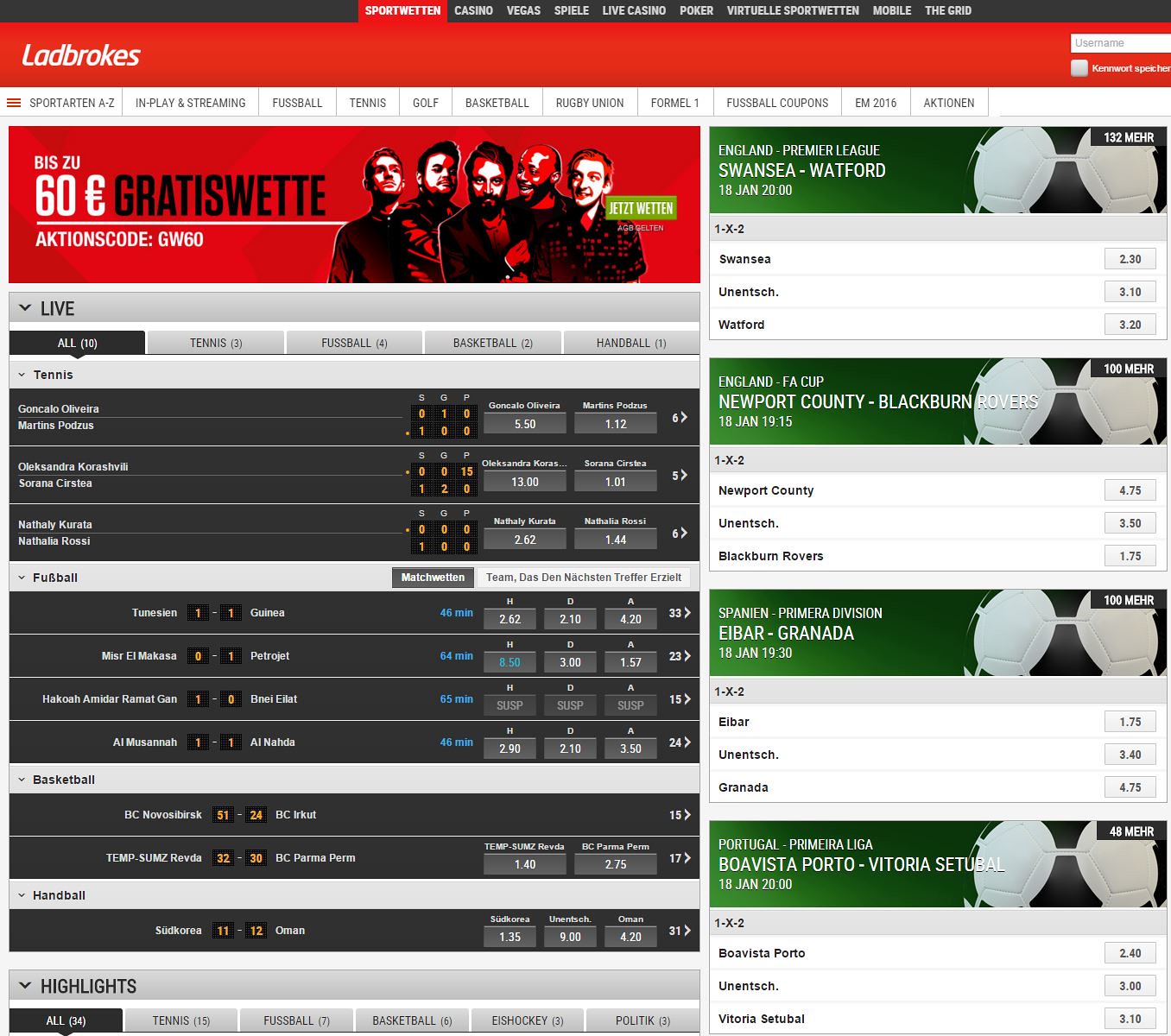This image is a detailed screenshot of a betting website that appears to be partially in German and English. At the very top, a black banner displays various options in white text, including "SportWetten," "Casino," "Vegas," "Spiel," "Live Casino," "Poker," "Virtual," "SportWetten Mobile," and "The Grid." Directly beneath this, a narrower red banner prominently shows the brand name "Ladbrokes" on the left side. Below this, a white stripe features black lettering with menu options such as "In Play and Streaming," "Fussball," "Tennis," "Golf Ball," "Basketball," "Rugby Union," "Forma One," "Fussball Coupons," and "EM 2016."

Further down the page, there is a red promotional banner displaying five men standing together, and the text "60 Euro G-R-A-T-I-S W-E-T-T-E" prominently next to them, indicating a promotional offer. The lower section of the screenshot contains black and green areas with various sports betting information and team names, some scores, and possibly ongoing or upcoming matches. There is a checkbox section for the username login along with other clickable box options scattered on the page. The monetary values are in Euros, highlighting its European audience. Overall, this screenshot captures a busy sports betting interface with a mix of promotional material and betting options.